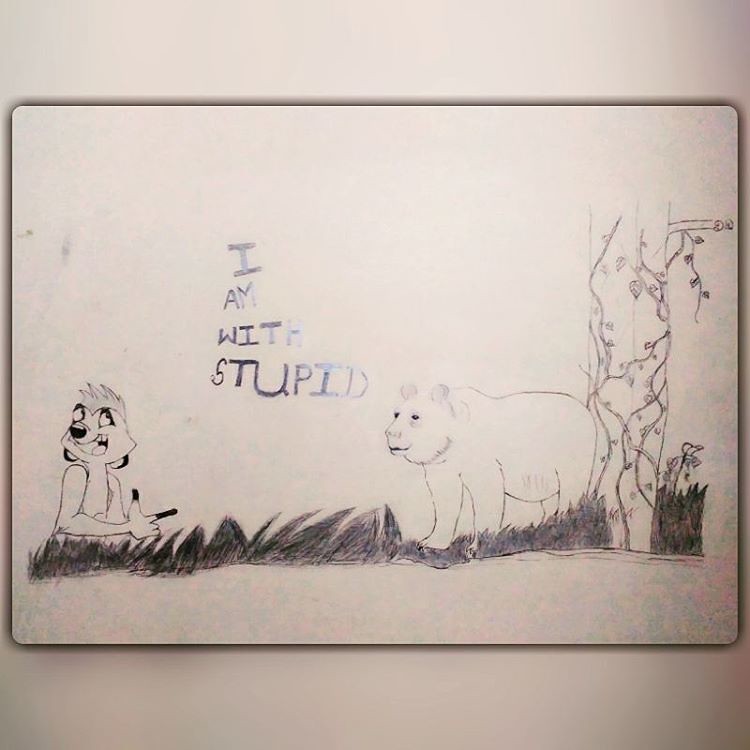This image is a black-and-white pencil drawing, characterized by a playful and whimsical style. On the left side, there is a cartoonish character that resembles either a fox or wolf. This character is depicted making a finger gun gesture directed towards the bear on the right. 

The bear in the image is lightly shaded, mostly white with a grayish-black outline, and is positioned near the center. Above the bear, the phrase "I AM WITH STUPID" is prominently displayed, with each word stacked vertically in all capital letters, filled with a gray tone.

A tree with intricately sketched vines climbing up its trunk stands behind the bear, providing a backdrop. The ground beneath the characters is illustrated with sparse, gray grass, adding texture to the scene.

The entire illustration is centered on a white piece of paper, which itself is placed against a white background. A subtle shadow border around the paper gives the drawing a floating effect. The overall composition creates a humorous and engaging scenario, brought to life by the detailed and expressive pencil work.